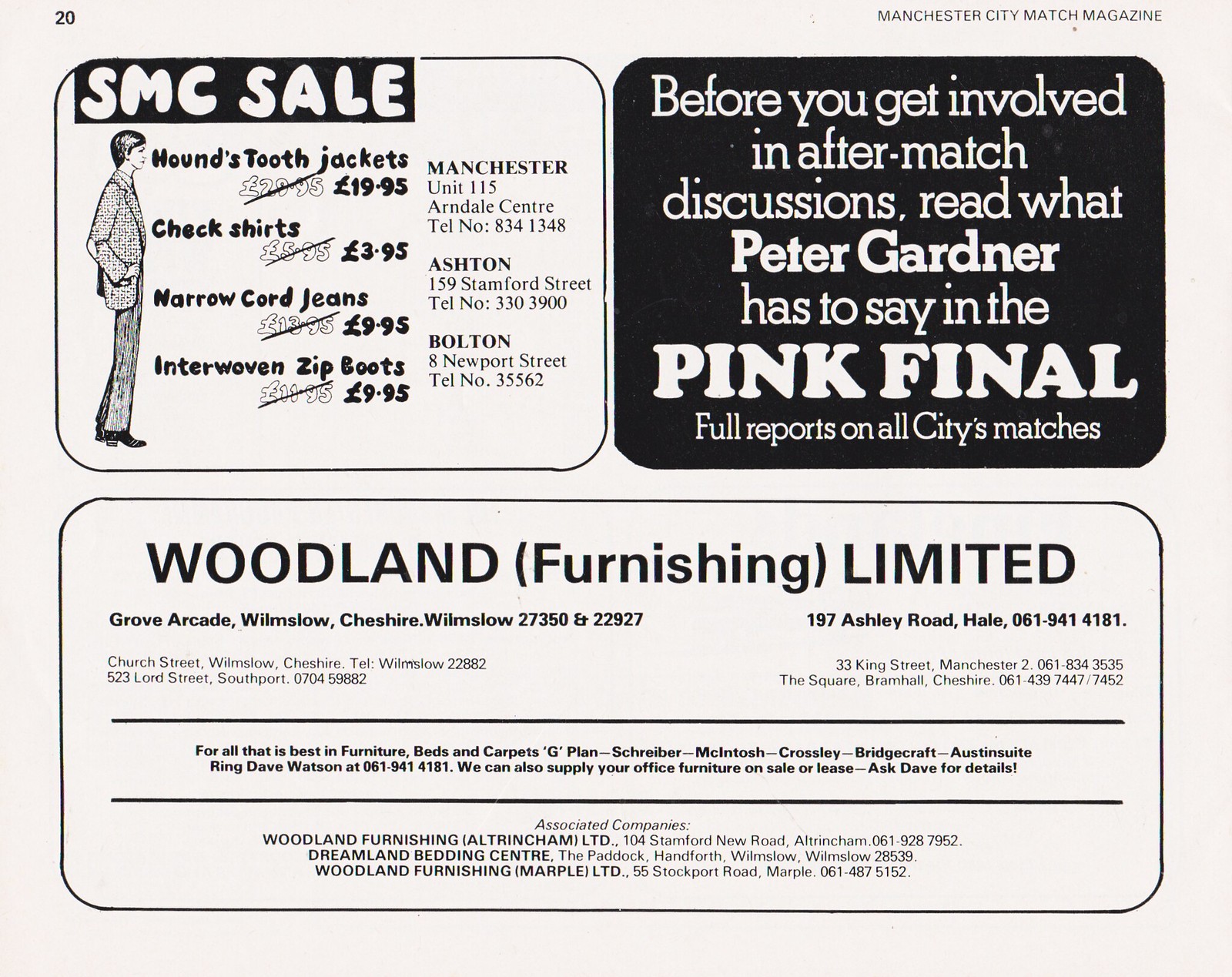The image is a horizontal magazine page numbered 20, featuring three distinct advertisements arranged in three sections. The top half of the page is split into two sections, while the bottom half consists of a single, wide section.

In the top left section, a white square with a black border houses a recognizable black banner with white text announcing "SMC Sale." Below this, in black lettering, several items and their prices are listed:
- Houndstooth jackets for £19.95 (€19.95).
- Check shirts for £3.95 (€3.95).
- Narrow cord jeans for £9.95 (€9.95).
- Interwoven zip boots for £9.95 (€9.95).

Additional information includes store locations and contact details:
- Manchester, Unit 115, Arndale Centre, Tel: 834-1348.
- Ashton, 159 Stanford Street, Tel: 330-3900.

The top right section, set against a black background with white text, invites readers to check out commentary by Peter Gardner in the "Pink Final" before engaging in post-match discussions. It promises full reports on all Manchester City matches.

The bottom half of the page is dedicated to an advertisement for Woodland Furnishings Limited, promoting high-quality furniture, beds, and carpets from brands such as G-Plan, Schreiber, McIntosh, Crossley, Bridgecraft, and Austin Suite. It also mentions that the company can supply office furniture for sale or lease, encouraging readers to "Ring Dave Watson at 061-941-4181" for details.

In summary, this magazine page effectively combines a variety of sales advertisements and informational content, aiming to attract a broad range of customers interested in fashion, sports commentary, and home furnishings.